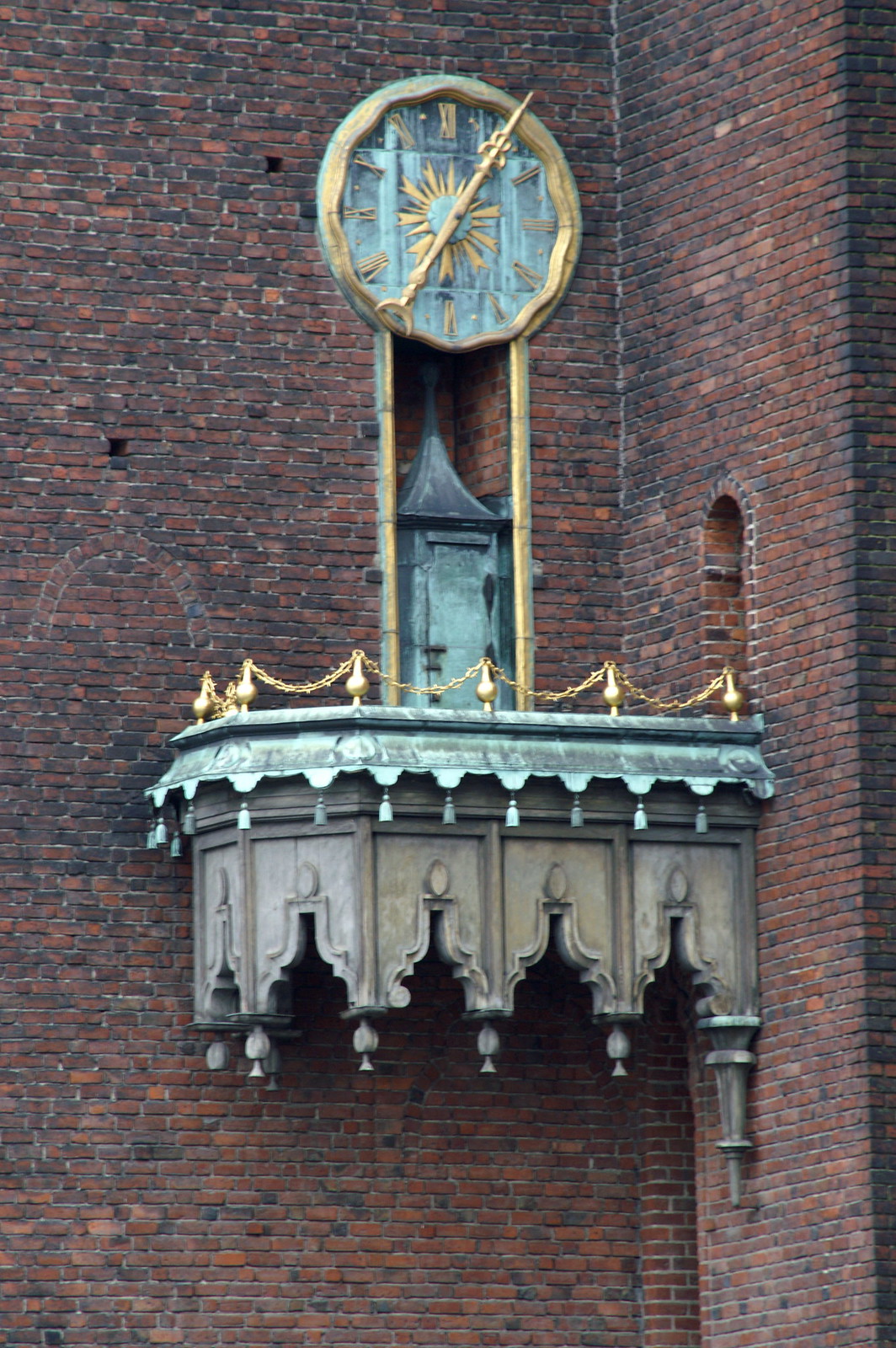The photograph captures a beautifully intricate antique clock mounted on the side of a building constructed from brown and gray bricks. The clock, notable for its large size, features a turquoise and blue face adorned with gold Roman numerals. Its scalloped edge is highlighted by a gold border, adding to its elaborate design. Below the clock is a small, closet-like structure with a dark blue, peaked roof and a turquoise-painted door, indicative of a functional space perhaps used for maintenance. This structure is positioned on a stone balcony, which includes carved details and a fence-like gold chain border. Accessible via an arched passageway in the brick wall to the right, the balcony allows individuals to walk out and admire the clock up close. The entire clock and balcony feature combine turquoise accents with gold and stone elements, creating a visually striking historical centerpiece on the building’s exterior.